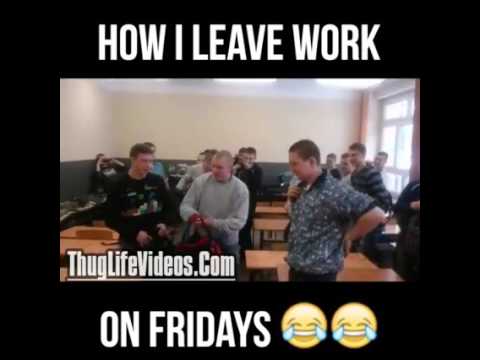The image is a meme featuring a black background with white text at the top reading "how I leave work on Fridays" and two laughing-crying emojis. In the center, there is a photograph of three young men in what looks like a classroom or office setting, with brown desks and bags on the table. The men are dressed casually – one in black on the left, one in gray in the middle, and one in a decorated shirt on the right who appears to be staring at the others. The man in the gray sweater seems to be putting on a backpack. Despite the text suggesting a work setting and the website thuglifevideos.com in the bottom left corner, the scene looks more like students leaving class, as the walls are half beige, half dark gray, with a window visible on the right side. The juxtaposition of the context and the casual demeanor of the men, who do not appear to be involved in any "thuggish" behavior, contributes to the humor of the meme.